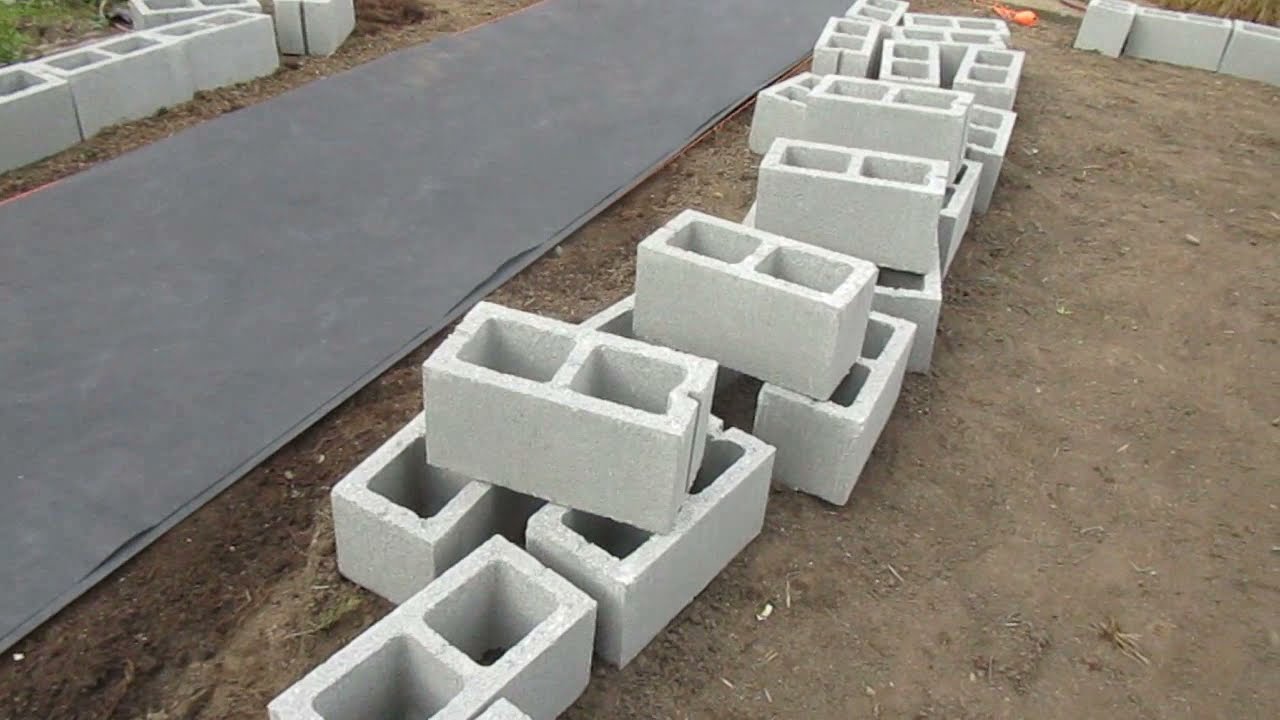The image depicts a construction site with a brown, compacted dirt ground. A dark gray or black fabric strip, resembling construction paper, runs diagonally from the bottom left to the top center of the photograph. Various cinder blocks, which are white or light gray in color, are scattered around the site. On the left side and in the background, they are stacked in rows, one layer high, suggesting initial stages of construction or temporary storage. Some blocks in the middle are mismatched and randomly placed. An orange string line is situated on the ground, adding a hint of ongoing construction activity. The scene is well-lit, indicating it was taken during the daytime.